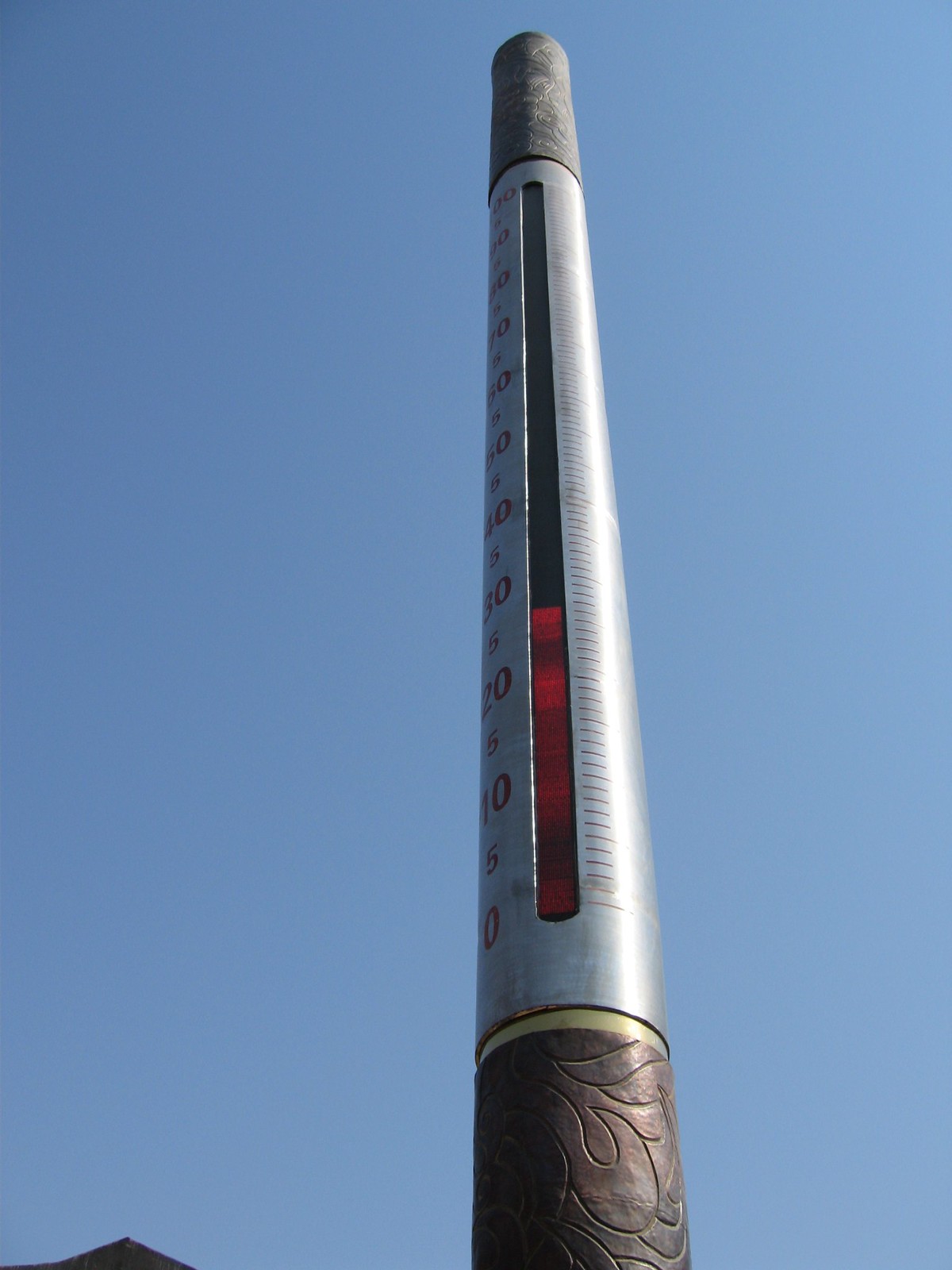The image depicts an elaborate, giant monument designed to resemble a thermometer. The structure is adorned with a decorative, floral-patterned, brown metallic base, which adds an artistic touch to its foundation. The primary feature of the monument is a central column that mimics the appearance of a traditional thermometer, partially filled with a deep red liquid that strikingly resembles blood. 

Along the length of the column, incremented numbers are clearly marked, starting at 0 and increasing by intervals of 5, specifically highlighting 0, 5, 10, 15, 20, 25, and 30. These numerical markers include halfway points, adding precision to the measurement display. Additional design elements, similar to those at the base, are present at the top of the structure, reinforcing its cohesive aesthetic.

The background of the drawing is a calm, solid blue, providing a neutral backdrop that contrasts with the vivid coloration of the thermometer-like monument. In the lower left corner of the image, there is a pointed structure, though its purpose and connection to the main monument remain ambiguous. It adds another layer of complexity and curiosity to the overall composition. 

This intriguing monument, blending functionality with artistic design, stands as a mysterious and detailed representation of measurement.